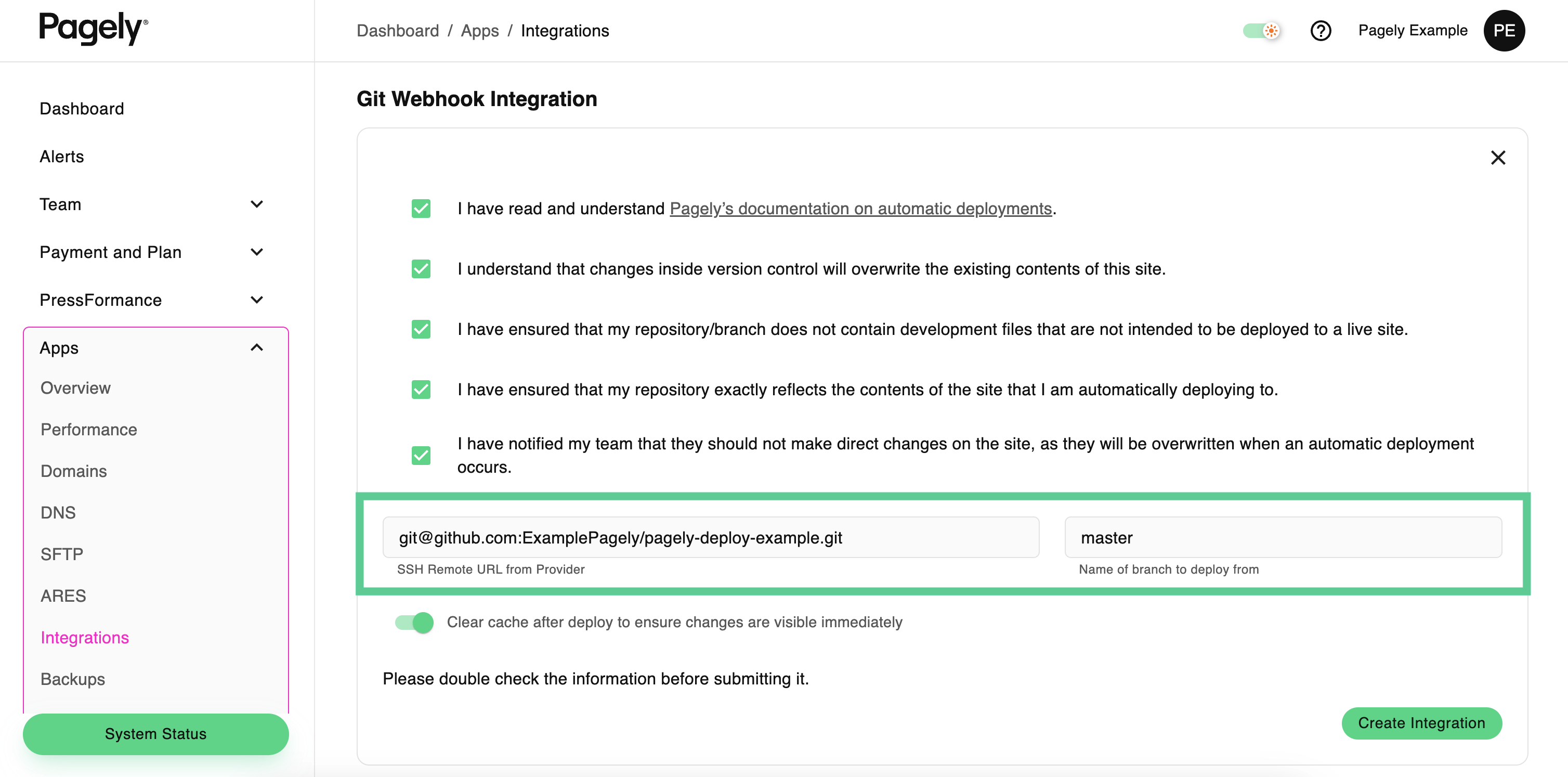The image is a screenshot of the Pagely website, which is designed for developing various web and computer applications. The page has a clean, white background with predominantly gray and black text. On the left side, a vertical navigation column provides information and access to different sections of the website. 

At the top of this column is the Pagely logo displayed in black text. Below the logo, several navigation links are arranged, offering access to various parts of the site, including the Dashboard, Alerts, Team, and Apps. The "Apps" link is highlighted with a pink border, indicating it is the currently selected section.

Within the "Apps" section, sub-options like Overview, Performance, and Integrations are available. The "Integrations" option is selected, with the text displayed in pink to show that it is the active page.

The central part of the page focuses on information about integrations for the app being developed. At the top center, the text "Git webhook integration" is prominently displayed in black, indicating that the current task involves setting up a Git webhook. 

Beneath this heading, there is detailed information about the Git webhook. This includes a series of checkboxes that the user must select to indicate they have read and agreed to the terms and conditions associated with the webhook setup.

Finally, in the bottom right corner of the image, there is a green button with black text that reads "Create Integration." Clicking this button will complete the process of creating the Git webhook for the application under development.